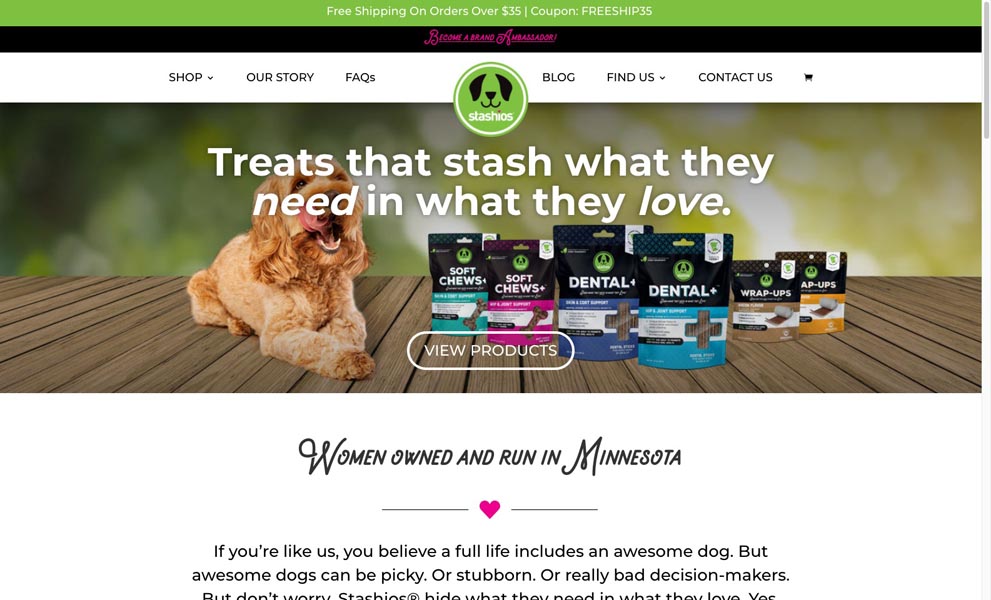**Website Description: Stashios - Premium Dog Dental Treats**

The screenshot is of the desktop version of the Stashios website, a company specializing in dog dental treats. Dominating the center of the webpage is an eye-catching photo banner featuring a medium-sized, poodle-like dog licking its lips, accompanied by several strategically placed, photoshopped bags of Stashios treats. These bags are labeled with product categories such as "Dental," "Soft Chews," and "Wrap-Ups." The banner's promotional tagline, highlighted in bold white text, reads: "Treats that stash what they need in what they love."

Prominently positioned below the banner is a call-to-action button labeled "View Products." The top navigation menu includes options such as "Shop," "Our Story," "FAQs," "Blog," "Find Us," "Contact Us," and a "Shopping Cart."

Immediately beneath the photo banner, a statement reads: "Women owned and run in Minnesota," adorned with a pink heart. This is followed by engaging text: "If you're like us, you believe a full life includes an awesome dog. But awesome dogs can be picky, stubborn, or really bad decision makers. Don't worry, Stashios hide what they need in what they love."

This detailed depiction effectively encapsulates the essence of the Stashios website, emphasizing both its product offerings and its user-friendly interface.